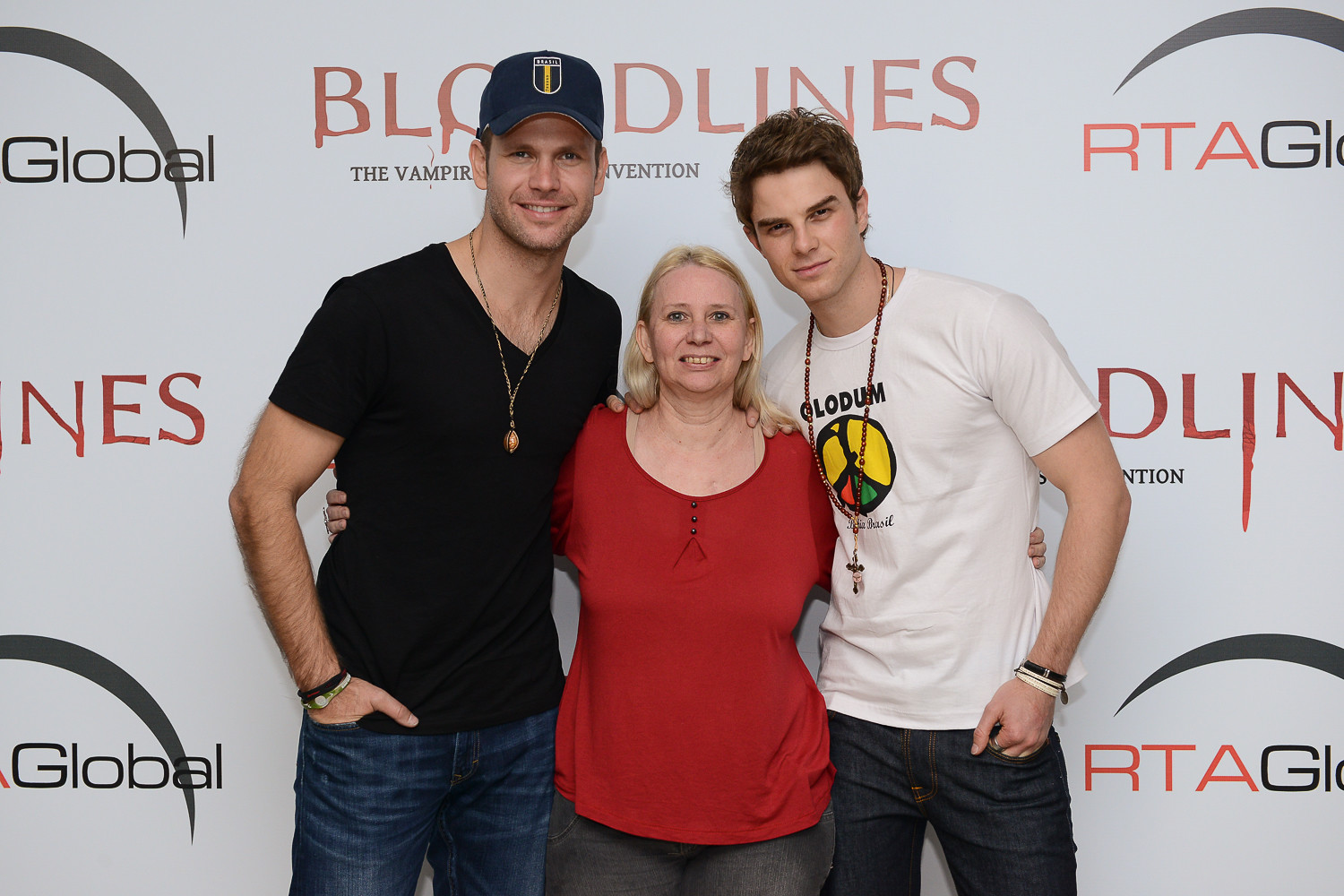This photograph captures a trio posing against a backdrop adorned with the logos "Bloodlines" and "The Vampire Convention," with additional text obscured by the central figure's head. The setting suggests they are on a stage or platform, likely part of a vampire-themed event. The group consists of two men and a woman. 

The man on the left is a tall individual in his 30s, wearing a blue cap, a black v-neck t-shirt, blue jeans, a gold necklace, a watch, and a bracelet on his right wrist. The woman in the middle, who appears to be in her 50s to 60s, sports a red blouse and black jeans; she has blonde hair. The man on the right, possibly in his 20s, has dark brown hair and is dressed in a white t-shirt, blue jeans, and a long necklace with a cross. All three individuals are posing confidently, suggesting their involvement or affiliation with the vampire convention.